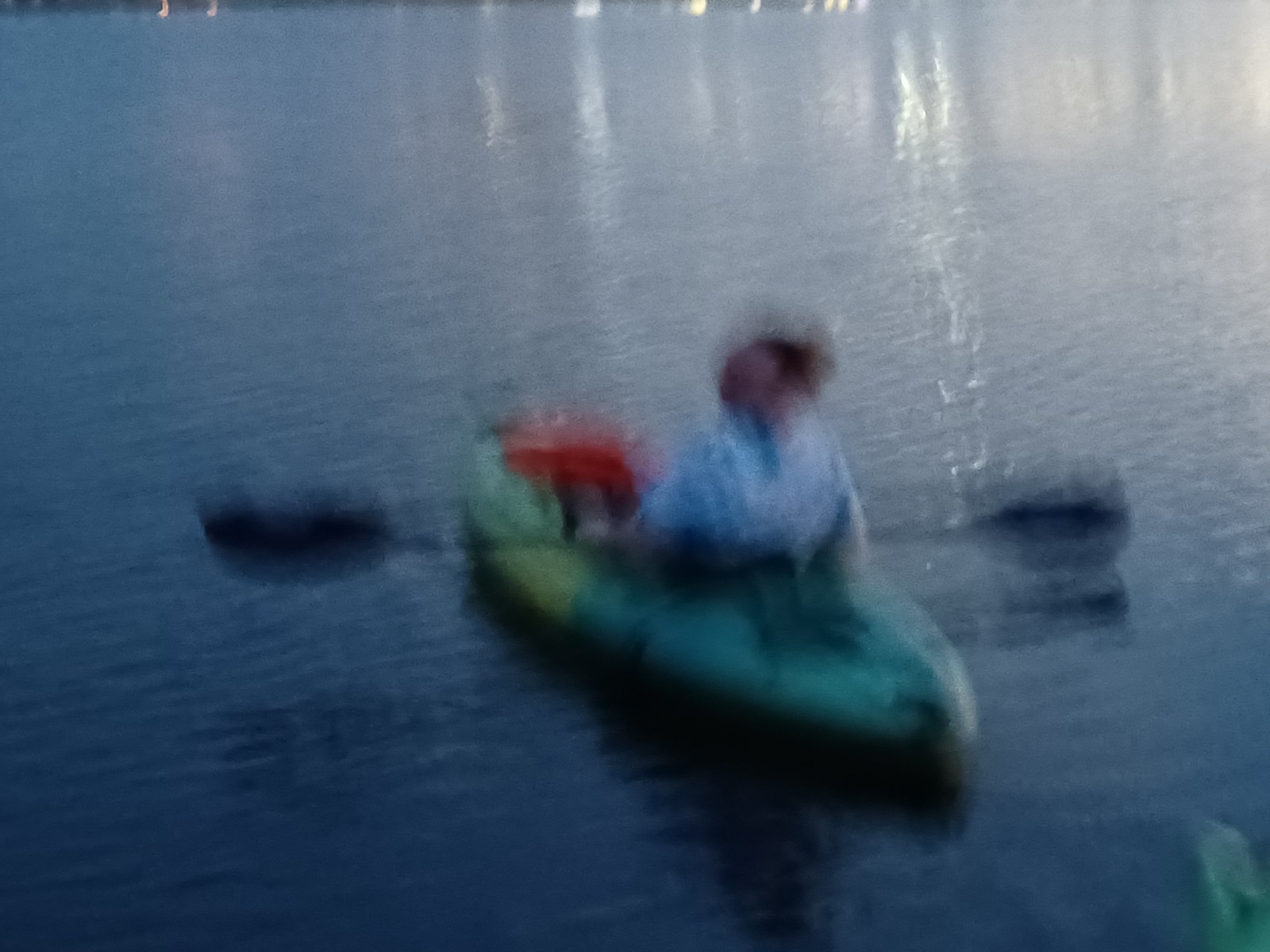This image is a very blurry photograph taken during what appears to be dusk or evening, featuring a person in a green kayak floating on water. The kayak, which seems to have a camouflage-like pattern with black and lighter green areas, is positioned diagonally in the frame with the rear end pointing towards the bottom right and the front towards the top left. The water is slightly rippled, possibly due to a long exposure time during the shot.

The person in the kayak is holding a black double-ended paddle across their thighs. They seem to be wearing a light-colored top, possibly white or blue, and are looking back towards the photographer. Unfortunately, due to the blurriness, it's difficult to discern the features of their face, but it appears darker in tone. There is a red object at the front of the kayak near their feet, though its exact nature is unclear due to the image quality.

In the distance, along the top edge of the photo, lights can be seen, possibly from the opposite shore, and their reflections shimmer in the water. The photograph's unclear and hazy quality suggests that it was taken with an unsteady hand and perhaps with a long exposure time, contributing to the overall blur and obscured details.